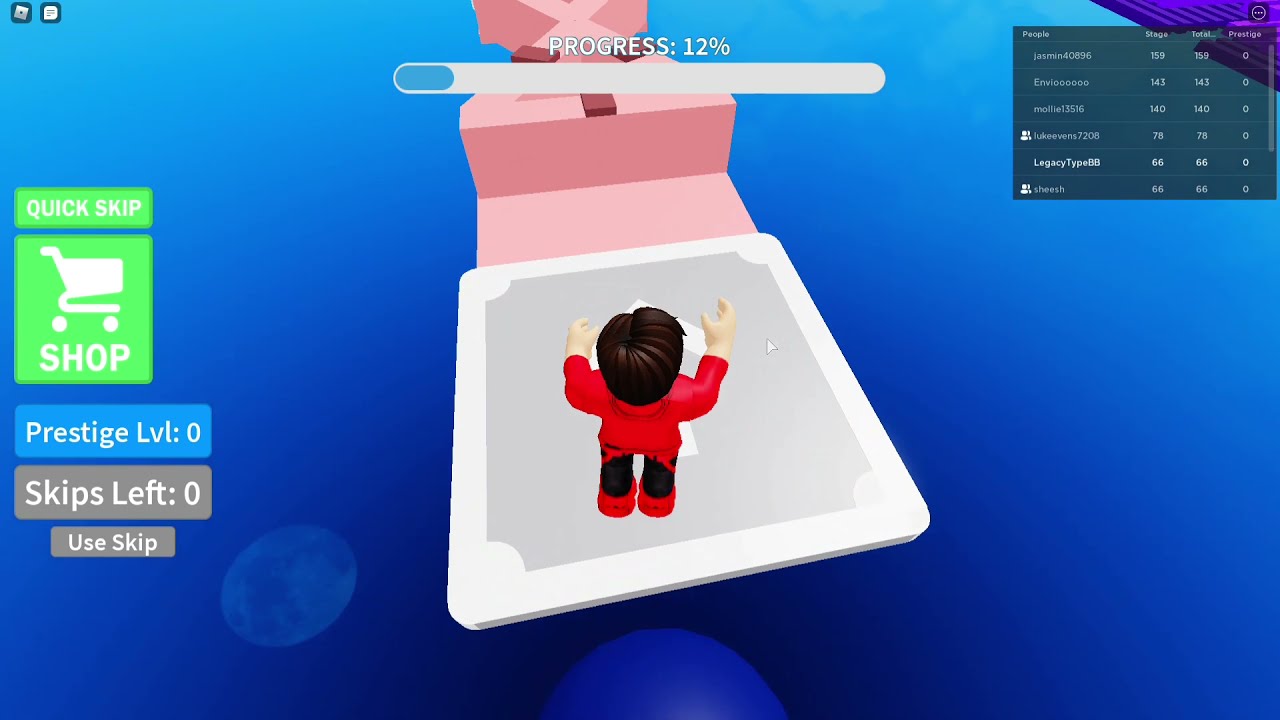This screenshot from a computer game features a vibrant blue background with a deep blue gradient at the bottom. A faint moon-like shape is visible on the far left side. At the center of the image is a large white square with a gray center, resembling a platform. On this platform stands a character with arms outstretched, wearing a red shirt, black pants, red shoes, and sporting brown hair. Directly in front of the white square is a pink platform with a sloped design that transitions to two triangular platforms. Above, a progress bar displays 12%. On the top right, various game stats can be seen, while the left middle section features icons and options labeled quick skip, shop, prestige level 0, skips left 0, and use skip. The setup and design suggest a whimsical game, likely geared towards younger audiences.